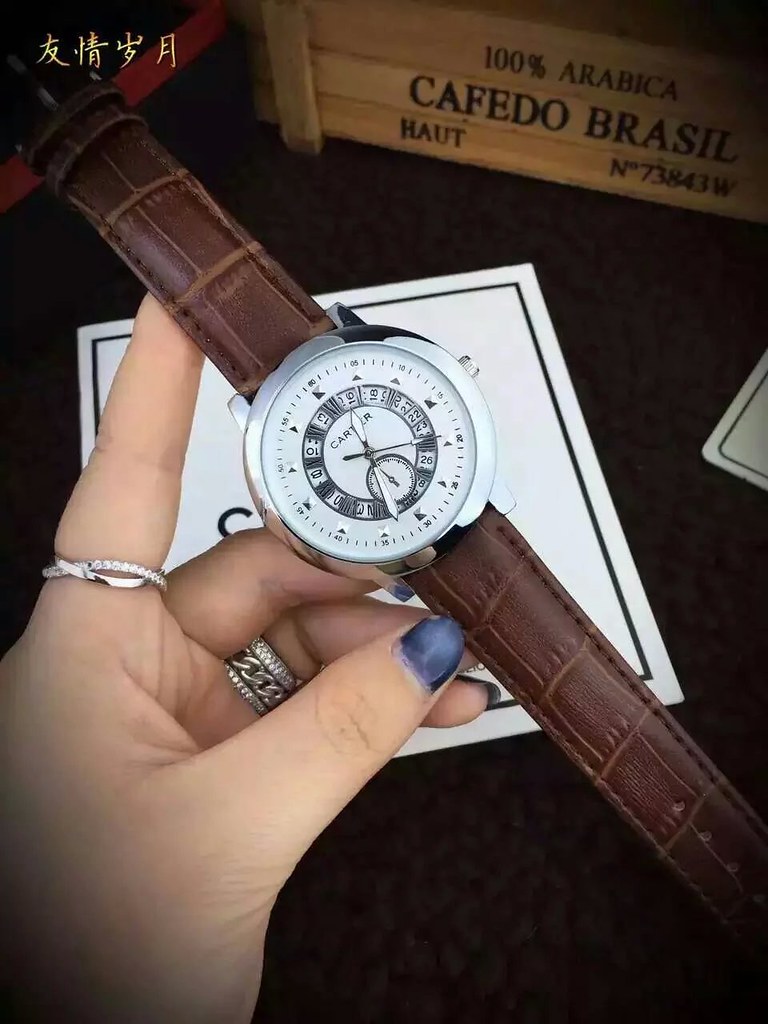In this photograph, a woman's hand, adorned with blue nail polish that's slightly chipped, showcases a luxurious Cartier watch. She is wearing a simple silver ring on both her index and ring fingers. The timepiece itself features a sophisticated brown alligator leather band. The watch's face is white and encased in what appears to be a silver metal, possibly silver steel or white gold, inscribed with the elegant "Cartier" logo. Adding to its opulence, the watch displays highly stylized Roman numerals that almost resemble intricate silver decorations. The hands of the watch are set to 1:33, completing this image of refined elegance.